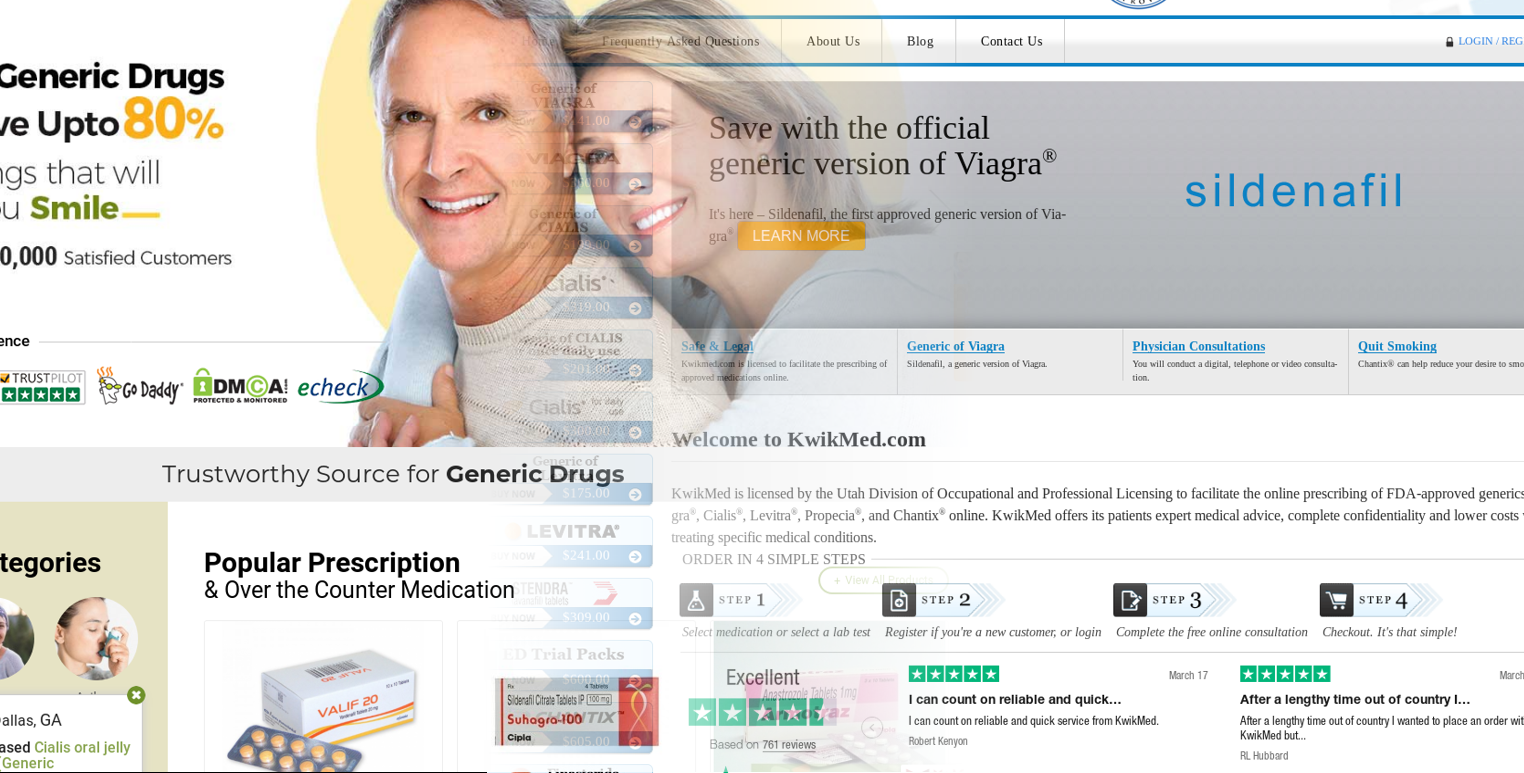The image shows a promotional page from a website, featuring a man and a woman. The man, positioned in the foreground to the left, has salt-and-pepper hair with subtle black streaks. Behind him, the woman, with her blondish-brown hair, affectionately wraps her arms around his neck and shoulders, resting her head gently against his. To the far left of the image, a banner reads "Generic drugs, save up to 80%, and that will make you smile." Part of the banner is cut off, obscuring the total number of satisfied customers mentioned. Below this, text promotes "popular prescription and over-the-counter medication," highlighting the "official generic version of Viagra" near the woman's head. The text appears overlaid, giving the impression of two images merged together. Towards the bottom of the page, the website's navigation invites users to explore various items, accompanied by a welcoming message: "Welcome to quickmed.com."